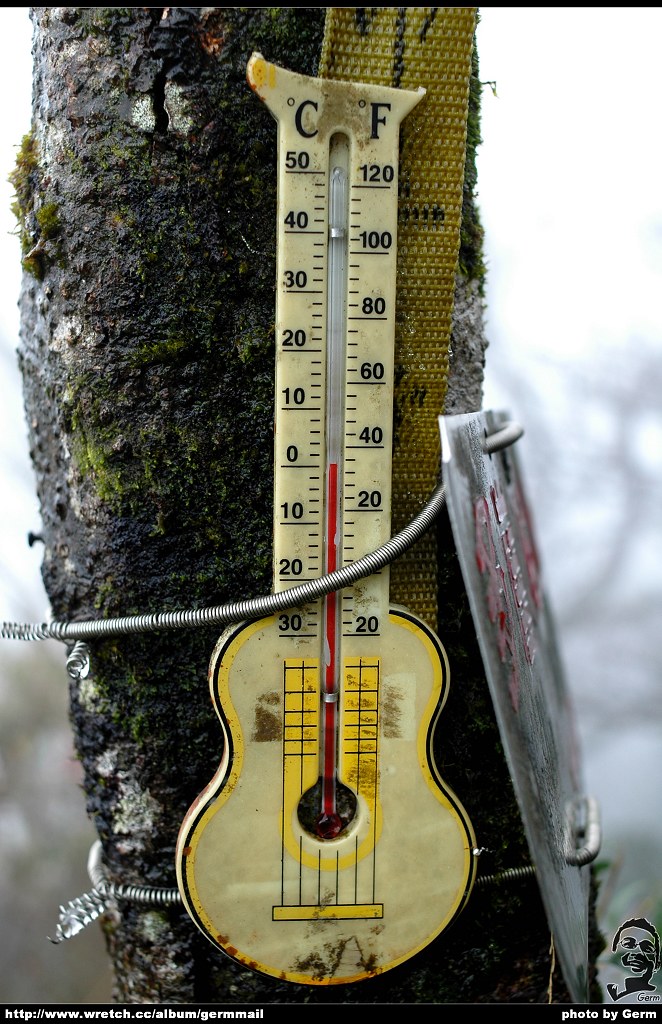A whimsical scene featuring a uniquely crafted door in the shape of a yellow guitar, weathered and faded from prolonged exposure to the sun, strapped securely to a tree. The temperature reads 35 degrees Fahrenheit (0 degrees Celsius), as indicated by a built-in thermometer on the structure. To the right of the thermometer, a piece of metal appears to serve as an anchoring mechanism, ensuring the guitar-shaped door stays upright. The entire contraption is held in place by thick, bracelet-like metal bands. The photo is credited to Germ, with a URL, retch.cc, mentioned on the left side.